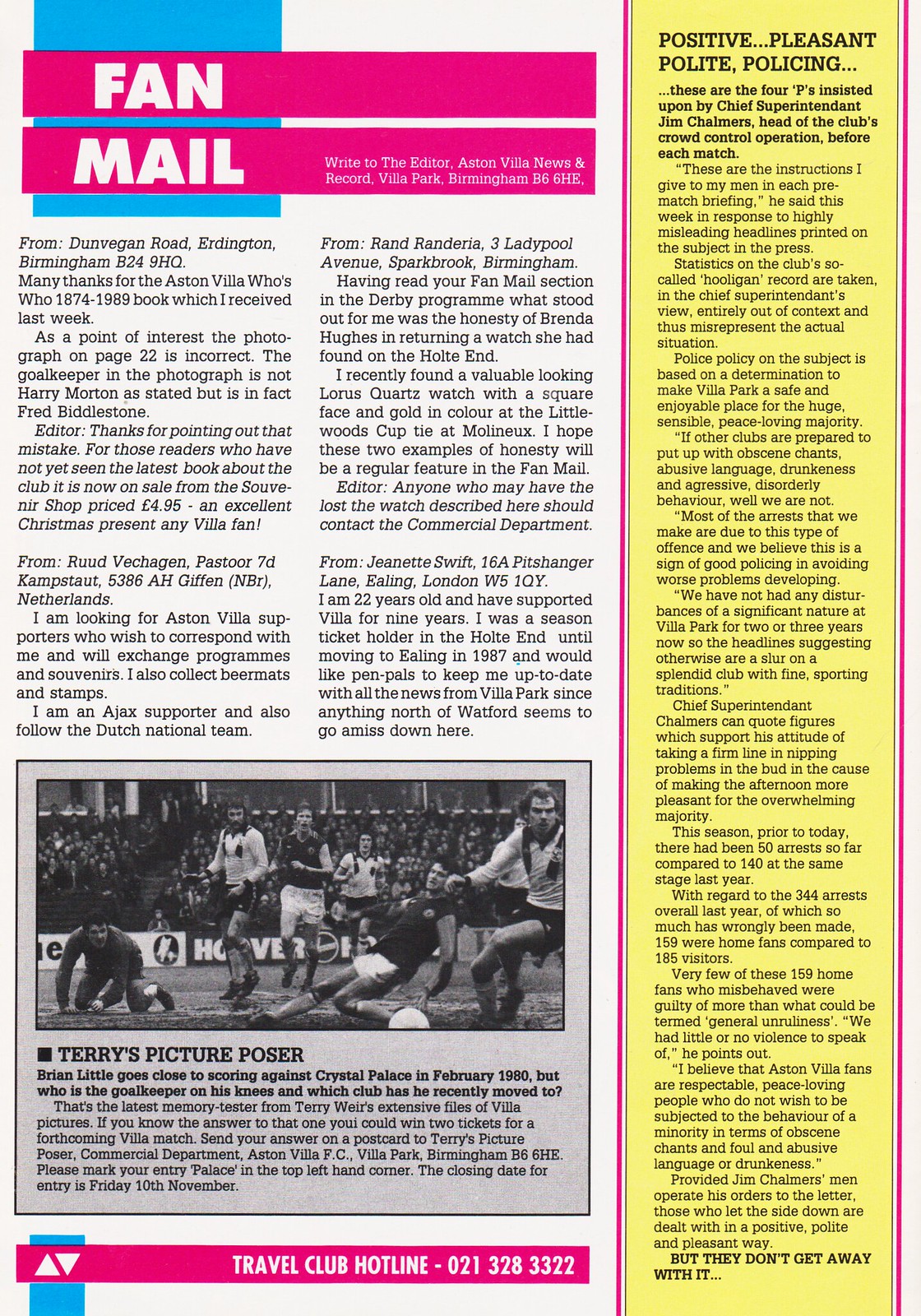This image is a detailed page from a magazine featuring fan mail and a soccer-related contest. On the left is a white background with structured text sections and a prominent photograph at the bottom. The top of the white section displays a blue square followed by two horizontal pink rectangles labeled "fan" and "mail" in white text. Below this, readers are encouraged to write to the editor at Aston Villa News and Record, Villa Park, Birmingham, B6 6888. The main content of this section includes letters from Aston Villa supporters. 

A letter from Ruud Vetschagen thanks for the Aston Villa Who's Who 1874-1989 book, pointing out a page 22 error where Fred Biddlestone is misidentified as goalkeeper Harry Morton. Another correspondent, Jeanette Swift, shares her desire for pen pals to keep her updated with Aston Villa news from Villa Park as she moved to Ealing in 1987. She commends Brenda Hughes for her honesty in returning a watch found at the stadium, and mentions finding a valuable Laura's Quartz watch herself, urging the owner to contact the commercial department.

At the bottom, the large black and white photograph captioned "Terry's Picture Poser" asks readers to identify a goalkeeper on his knees, during a match where Brian Little almost scores against Crystal Palace in February 1980, offering a prize for correct answers. 

On the right, a narrow yellow column titled "Positive, Pleasant, Polite Policing" emphasizes the club's focus on ensuring a safe and enjoyable environment at Villa Park. Chief Superintendent Jim Chalmers outlines the firm and respectful policing strategies aimed at minimizing disturbances and providing a positive atmosphere for the majority of the fans. He defends their record against misleading press claims, highlighting a significant reduction in arrests compared to the previous year. 

Overall, the page combines fan interactions, community spirit, and the club's dedication to maintaining a disciplined but pleasant stadium experience.